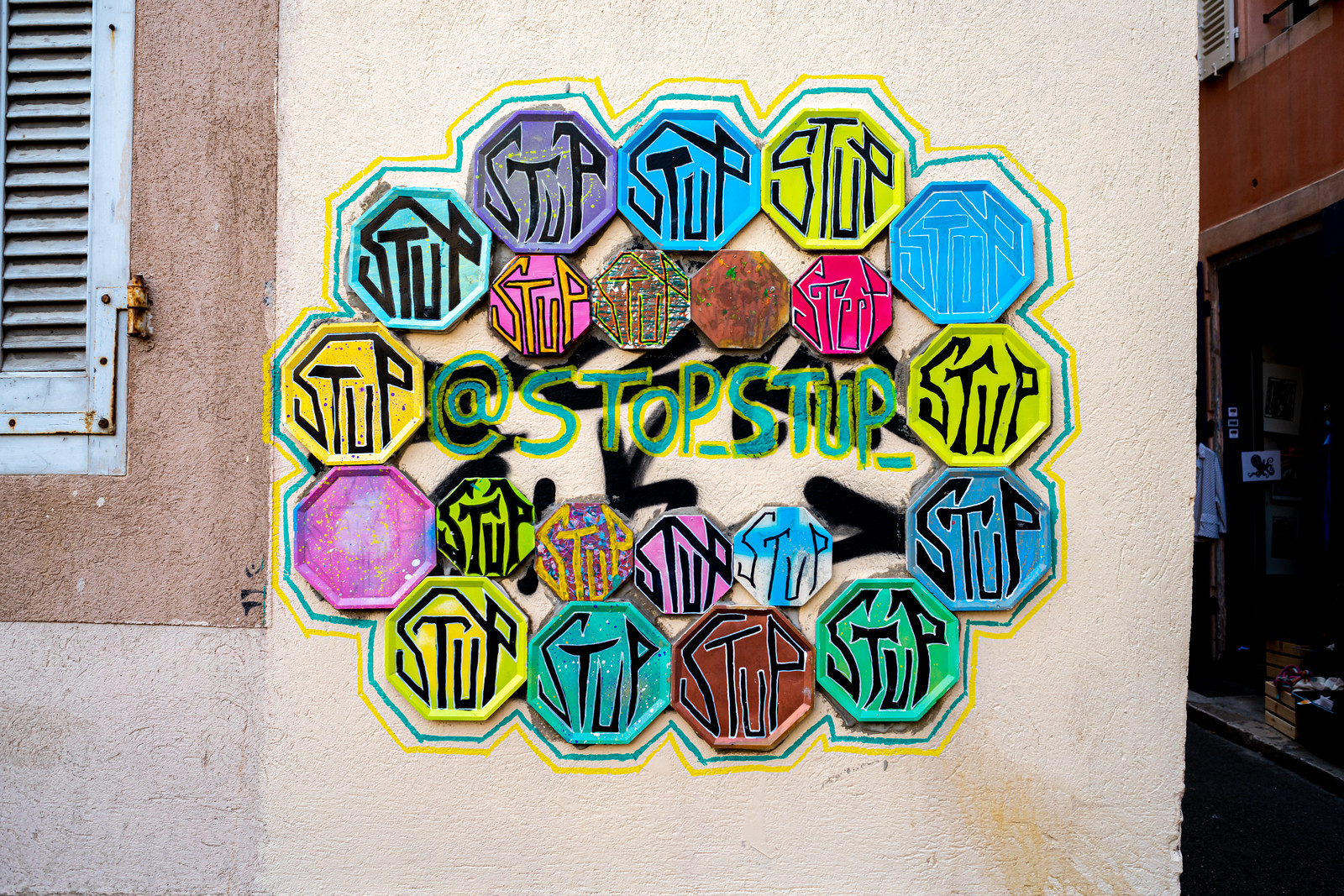The detailed mural painted on the cream-colored, plastered wall at the edge of a building represents a collage of octagon-shaped images reminiscent of stop signs. Each octagon is distinct, showcasing a variety of vibrant colors including greens, browns, blues, purples, and more, with the word "STUP" prominently displayed in either black or blue letters. At the center of the mural, the phrase "@stop_step_" is highlighted in green with yellow accents, encircled by a series of smaller octagon shapes. These smaller octagons echo the central theme and design, creating an intricate pattern that forms a large circle around the centerpiece. This elaborate street art blends seamlessly with the surrounding environment, which includes a two-toned wall on the left and a dark street scene on the right, partially visible alongside the mural.